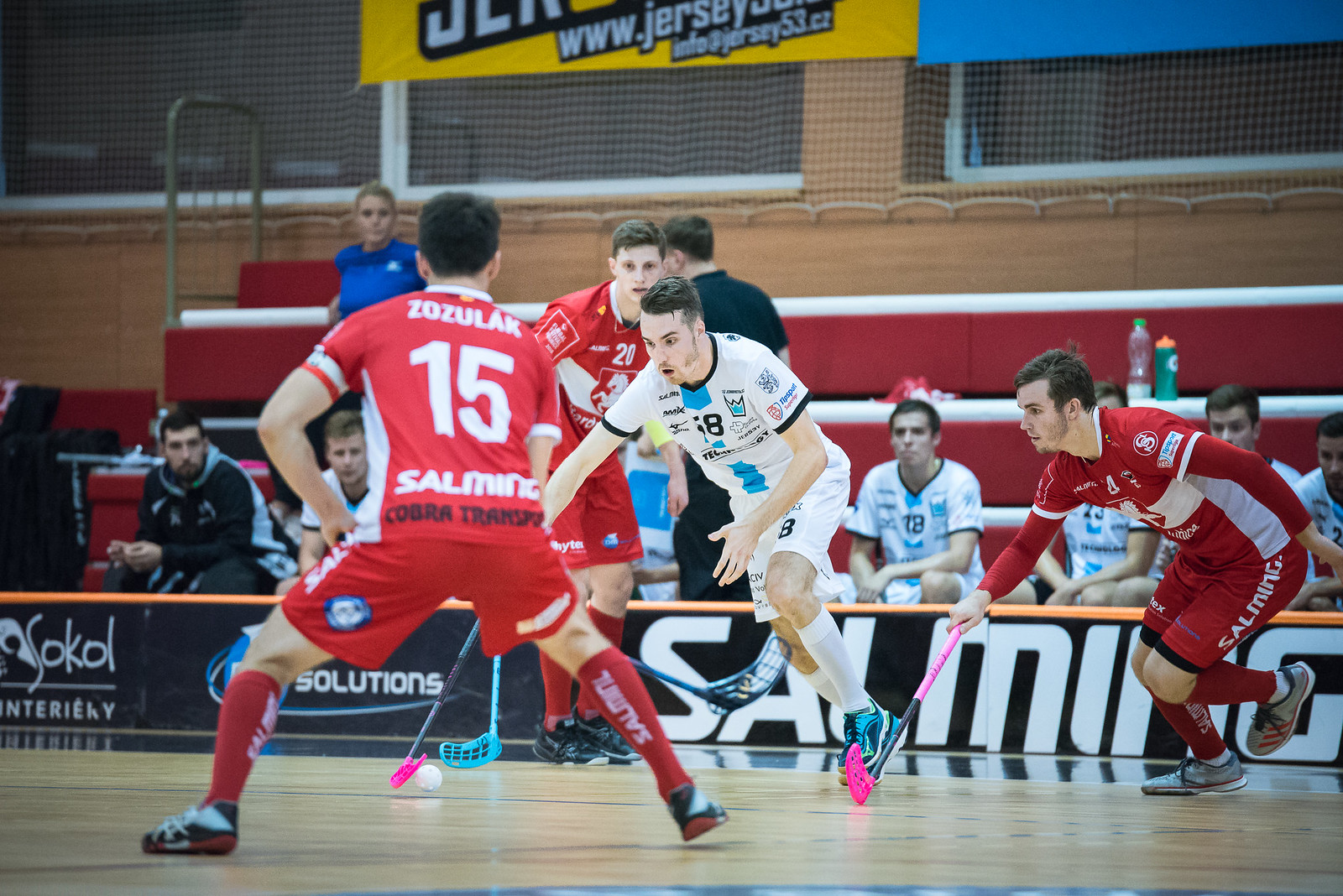A detailed photograph captures an intense floor hockey game in an indoor stadium. The white team, led by a player dressed in a white short sleeve shirt, white shorts, white high socks, and blue sneakers, is in control of the ball while facing off against three players from the red team. The red team players are clad in red and white short sleeve shirts, red shorts with white lettering, and red high socks with sneakers. In the background, a low wall separates the playing area from the spectators, where team members from the white team are seated and watching the game. Additionally, there are three individuals in casual attire, two standing and one sitting, observing the match. While the stands are not completely full, a few people, likely coaches and substitutes from the white team, are present. Behind the teams, a partially visible sign reads "info at jersey53.cz" with the sponsor name "SOKOL" discernible, suggesting possible Polish and Czechoslovakian connections. The game, featuring prominent red, white, and black team colors, appears to be part of a competitive sports event.